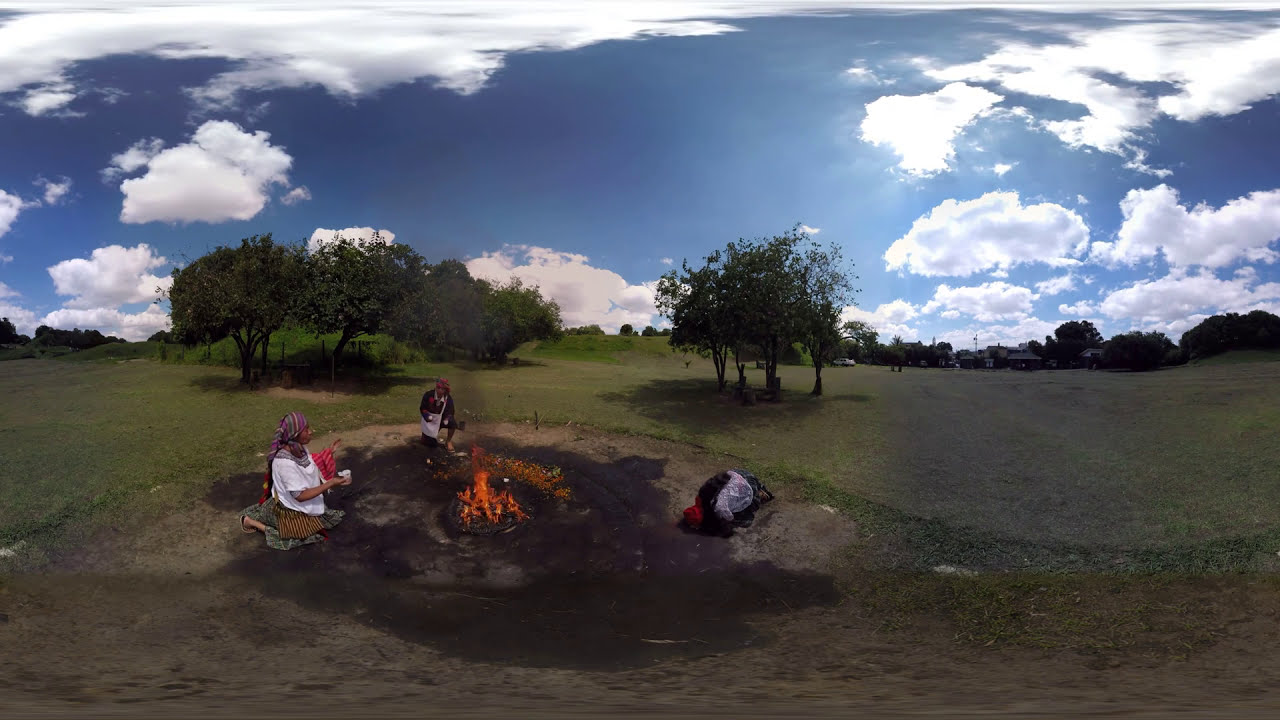In the center of the image, there is a lit bonfire situated on a grassy surface, slightly towards the bottom left. Surrounding the bonfire are three African American women dressed in traditional African attire. One woman is kneeling to the left of the fire, another is positioned behind it, and the third woman, to the right, appears to be bowing in prayer. The setting is an outdoor, open field under a partly cloudy sky, with visible blue, white, gray, green, orange, yellow, purple, tan, and black colors. The ground directly under and around the fire is scorched, indicating recent activity. Beyond the immediate scene, there is a grassy field extending to the horizon, scattered with a few trees and a distant hill. On the right side of the photo, a silver and black backpack is placed near the women, and farther in the background, two people can be seen walking several hundred yards away. Additionally, a white car is parked alone off to the right, and some buildings are faintly visible in the distance. The overall ambiance suggests a serene midday gathering in a cleared-out area.